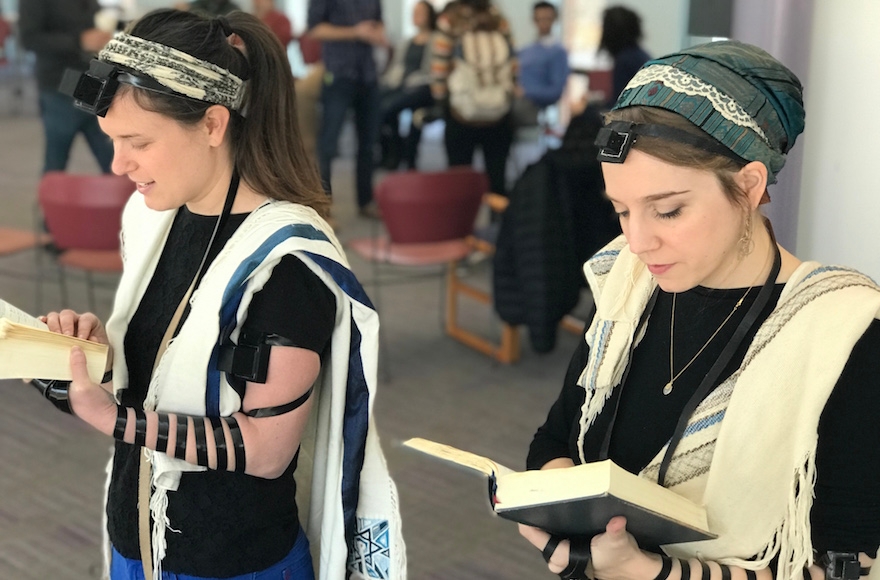In the photo, two women are standing indoors, appearing to be engaged in an Orthodox Jewish ritual. They are reading from an open book, with most of the book seemingly read from the right side, as characteristic of Hebrew texts. Both women are wearing black tops and distinct garments, which resemble traditional Jewish prayer shawls with the Star of David on them. On their heads, they wear distinctive items – one with a bandana and her hair in a ponytail, and the other with a headdress and a necklace. They both have black phylacteries (tefillin) attached to their foreheads and wrapped around their left arms. The background reveals a blurred circle of people, with discernible red chairs and a black jacket hanging on one.